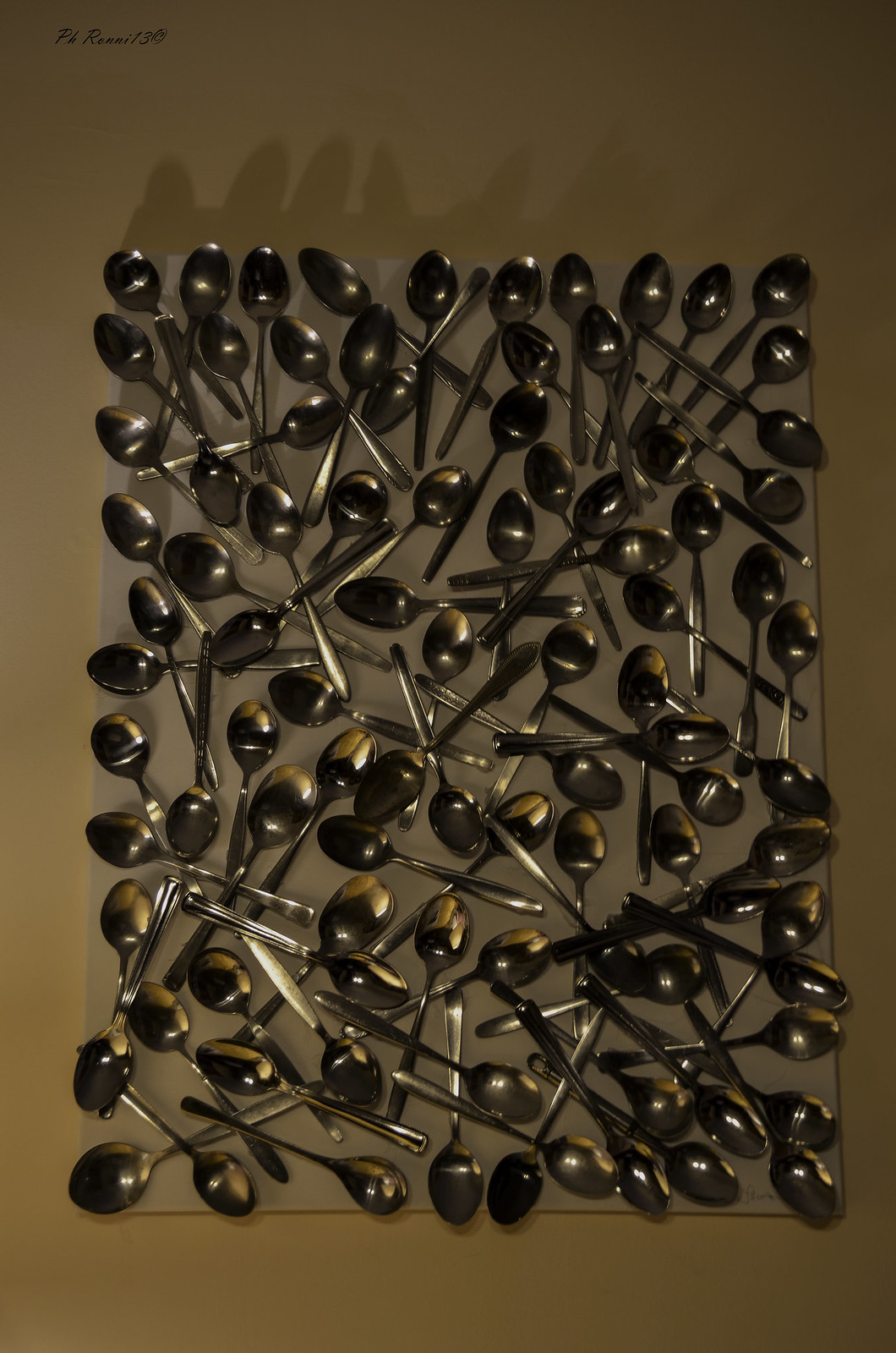This photo captures an artistic arrangement of approximately a hundred silver spoons, displaying an intricate play of light and shadow. The spoons, varying in orientation and occasionally overlapping, are meticulously laid out on a slate-gray background, which further enhances their reflective surfaces. Some spoons reflect a warm golden hue, creating an impressive contrast against the predominantly dark tones of the metal. Each spoon's position and tilt—left, right, up, and down—add to the dynamic visual interest, casting shadows that contribute to the overall texture of the image. This captivating collection of spoons resides within a lighter gray frame, suggesting it might be mounted on a wall, possibly with the spoons glued in place. In the top left-hand corner, a name is inscribed, potentially signifying the artist or photographer. The deliberate randomness and reflective quality of the spoons give this artwork its unique elegance.